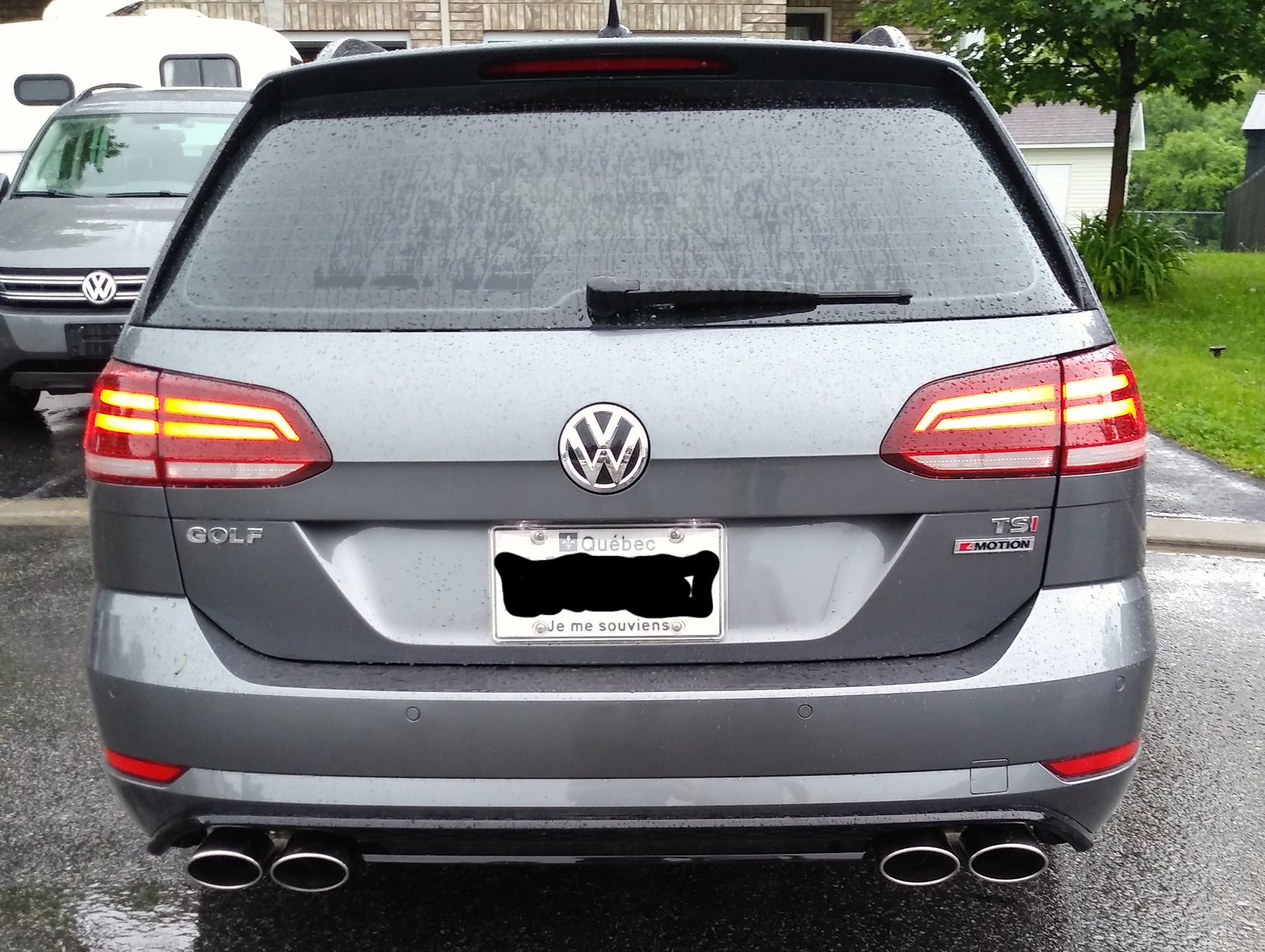This detailed photograph captures a close-up view of the back end of a gray Volkswagen Golf on a rainy day. Water beads on the car's surface and streams down the back windshield, which features a wiper blade that is not in use. The brake lights are lit up in red with a hint of yellowish glow. The vehicle sports distinctive badging with "Golf" on the left and "TSI eMotion" on the right. Notably, four silver exhaust tips are visible—two on each side.

The license plate, indicating that the car is from Quebec, Canada, reads "JE ME SOUVIENS." Parked in a residential area, the car is positioned near a garage, with a camper and another Volkswagen nearby. The setting includes beige and cream-colored brick on the house, a nicely landscaped yard with a well-maintained lawn, a tree, and some greenery. A small white shed is also visible off to the side. The silver roof rack on the car hints at its readiness for travel or additional storage. The overall scene exudes a quiet, rainy day in a well-kept neighborhood.